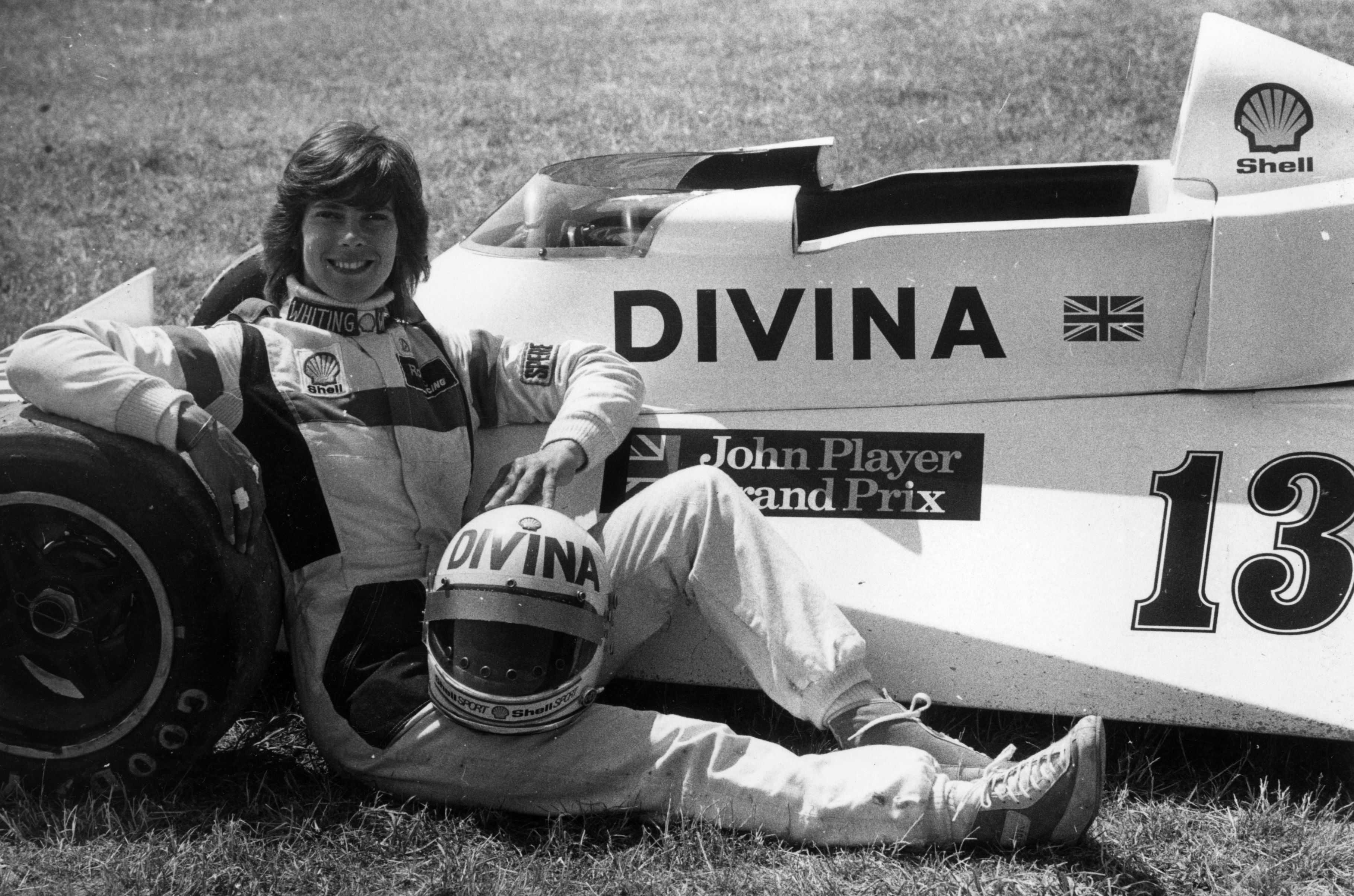In this detailed black-and-white close-up photograph, a woman named Divina is seated in a grassy field next to a small, roofless race car. She is dressed in a distinctive race uniform that is predominantly white with black stripes, featuring the Shell gas station logo on the right breast and the name "Whiting" near the collar. The uniform extends down to her ankles, and she pairs it with tennis shoes with white laces, resembling Converses. Divina, who has short shaggy brown hair with bangs, is smiling warmly as she leans her right elbow on the front driver’s side tire of the car. Her helmet, inscribed with "Divina" in black letters, rests on her lap. The car, which is white with a small plexiglass windshield above the steering wheel, prominently displays "John Player Grand Prix," the number 13, the Shell logo, and the name "Divina" on its body. A British flag can also be seen among the decals. The scene is set outdoors during the day, capturing a moment of poised relaxation and pride.